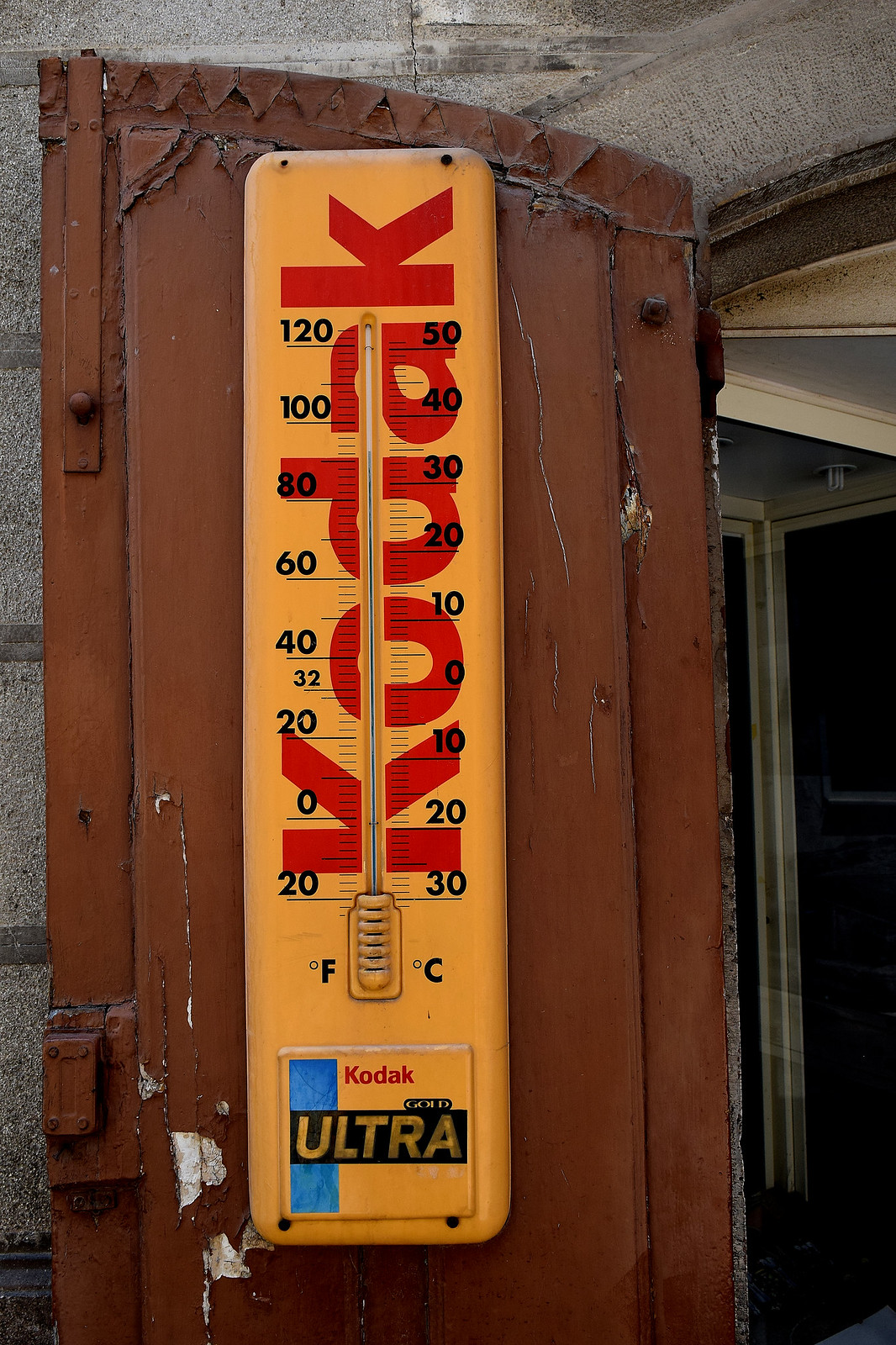This outdoor photograph captures a nostalgic Kodak thermometer, standing prominently at two to three feet tall with a rectangular, vertical shape. The thermometer features a vibrant golden-yellow background with the brand "Kodak" emblazoned in red font. A glass mercury gauge runs through the word "Kodak," meticulously marking temperature in both Fahrenheit and Celsius.

On the Fahrenheit side, numbers are displayed from top to bottom: 120, 100, 80, 60, 40, 32 (in a smaller font), 20, 0, and -20, with shorter and longer dashes in between each number for precise measurement. Next to each Fahrenheit number, an icon "°F" marks the unit.

The Celsius scale on the opposite side lists: 50, 40, 30, 20, 10, 0, -10, -20, and -30, similarly accompanied by corresponding dashes for accuracy.

Beneath the thermometer, a square section prominently featuring the Kodak name again, this time with the word "Ultra," reminiscent of the design found on a box of Kodak film.

This charming thermometer is firmly mounted on a rustic, brown-painted wooden door, adding a touch of timeless vintage character to the outdoor setting.